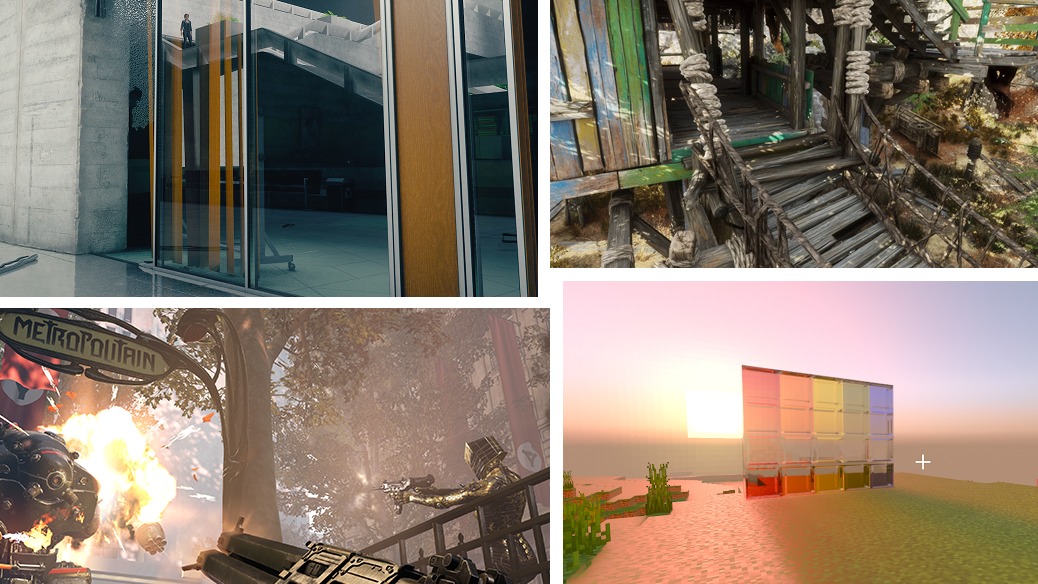The image is a composite of four distinct sections, arranged in two rows. The top left section features a highly reflective window on the side of a building, capturing a man standing on a staircase inside. This scene might be a digital drawing. Below this, a scene set under a tree shows a man wearing a metal outfit firing a weapon, with an explosion to the left and a small fence in the background. Moving to the top right, there's an image of a dilapidated wooden structure painted in faded blue and green hues. The structure has an open doorway leading to a bridge made of weathered wood, with ropes holding the poles together. Finally, the bottom right section displays a series of vividly colored panels arranged in rows, with colors ranging from red, orange, yellow, green, to blue, possibly representing the sides of shipping containers or another patched-together screen, set against a desert backdrop.